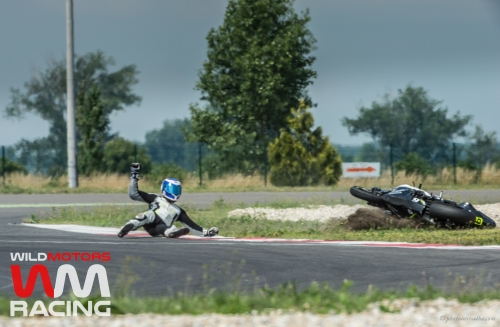The image captures a motorbike accident on an asphalt racetrack, showcasing a detailed mid-slide moment of the rider. The rider, dressed in a racing outfit with a white chest, gray and black sleeves, and matching pants, is equipped with special boots and a complete helmet with a tinted blue visor. They are sliding on their left side with no bike underneath them. The black motorbike, turned over on its side, has black wheels, part of the left handlebar visible, and a yellow sticker. The track, marked by a logo that says 'Wild Motors WM Racing' in red and white on the left-hand side, is surrounded by green leafy trees and a mostly gray sky above. In the distance, a sign with a red arrow points right, adding to the scene's racing ambiance.